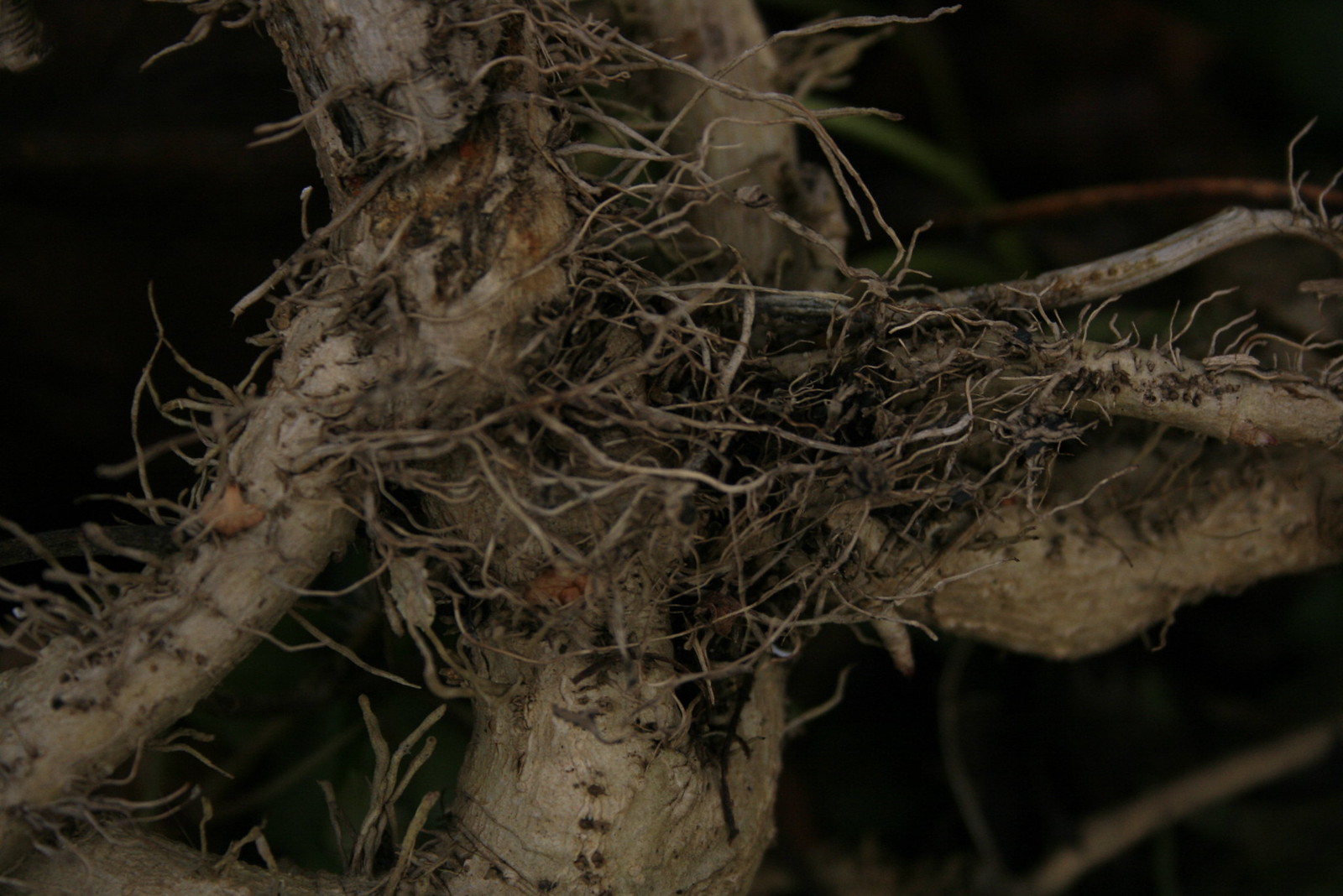This is a detailed photograph capturing a close-up view of what appears to be part of a tree, possibly a tree trunk or a root system. Central to the image is a prominent branch or trunk that stretches vertically, with several thinner, root-like or stringy branches extending outward to the left and right. These secondary branches seem cracked and fragile, giving an impression of decay or wear, likely influenced by insect activity. The insects might have used the material to construct a nest, as suggested by the presence of pulp and a nest-like structure integrated into the wood. The primary structure is a grayish-white color with darker, almost black, recesses, and lighter beige elements. The background is out of focus, displaying blurred streaks of green and brown, possibly indicating leaves and other parts of the tree. This environment suggests a dark, green setting, and the photograph appears to have been taken in low lighting, emphasizing the detailed textures of the branches and roots against a subdued backdrop.